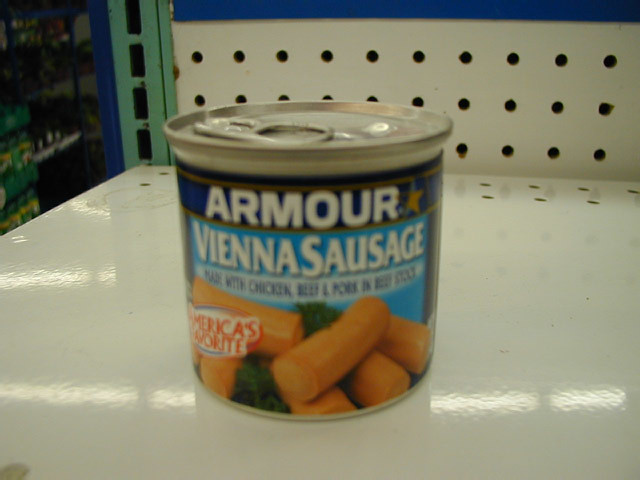A can of Armour Vienna Sausage is prominently displayed in the foreground. The label indicates that it is made with chicken, beef, and pork, proudly proclaiming itself as "America's Favorite." The can rests on a white surface, resembling a shelf. To the left, there is another section of shelving filled with various items. The background features a pattern of black holes, adding depth to the scene. On the far left shelf, there's a splash of green. Nearby, English text in black is visible, providing additional information.